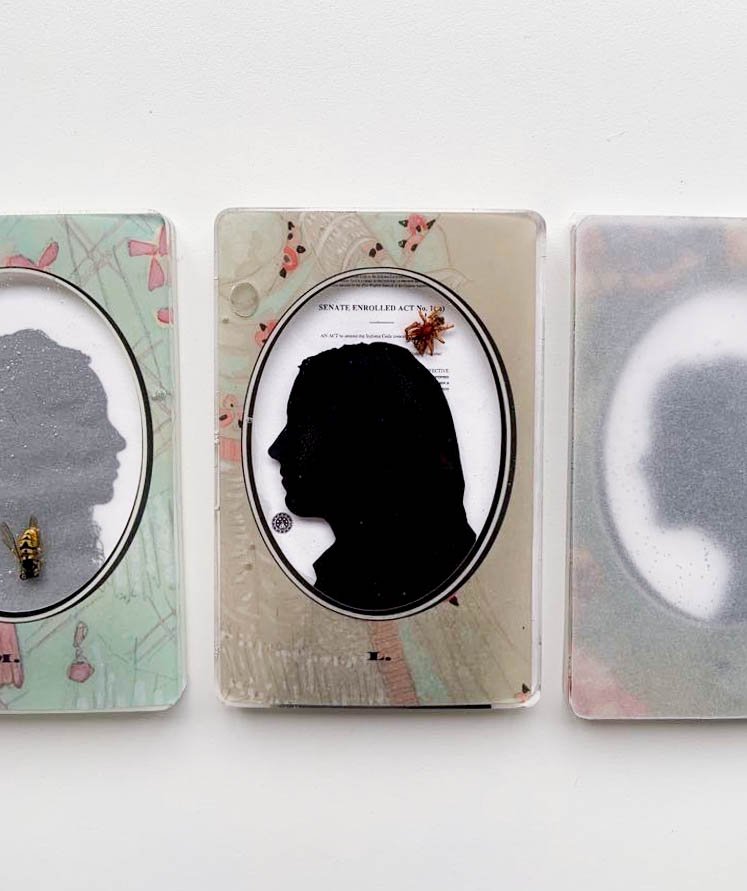This photograph showcases three framed silhouettes of female profiles, each uniquely encased in square, cassette-sized plastic frames with oval cutouts. The left frame features a light green border adorned with faint pink floral patterns and a prominent dead yellow jacket bee perched on the black silhouette of a girl with long hair, which is slightly hazy. The central frame, the most vivid and clear of the trio, is tan with touches of pink and green scribbles, almost resembling dried flowers embedded within the resin. This frame contains a black silhouette of a girl with her head held high, overlaid with a translucent document bearing the word "Senate," and a smashed spider. The right frame, enveloped in a protective rice paper, appears muted and indistinct, revealing only the general shape of a black silhouette against an unclear backdrop. These trinkets collectively present an intriguing blend of delicate colors, floral decorations, and unexpected details like insects, encapsulating an ethereal yet eerie aesthetic.